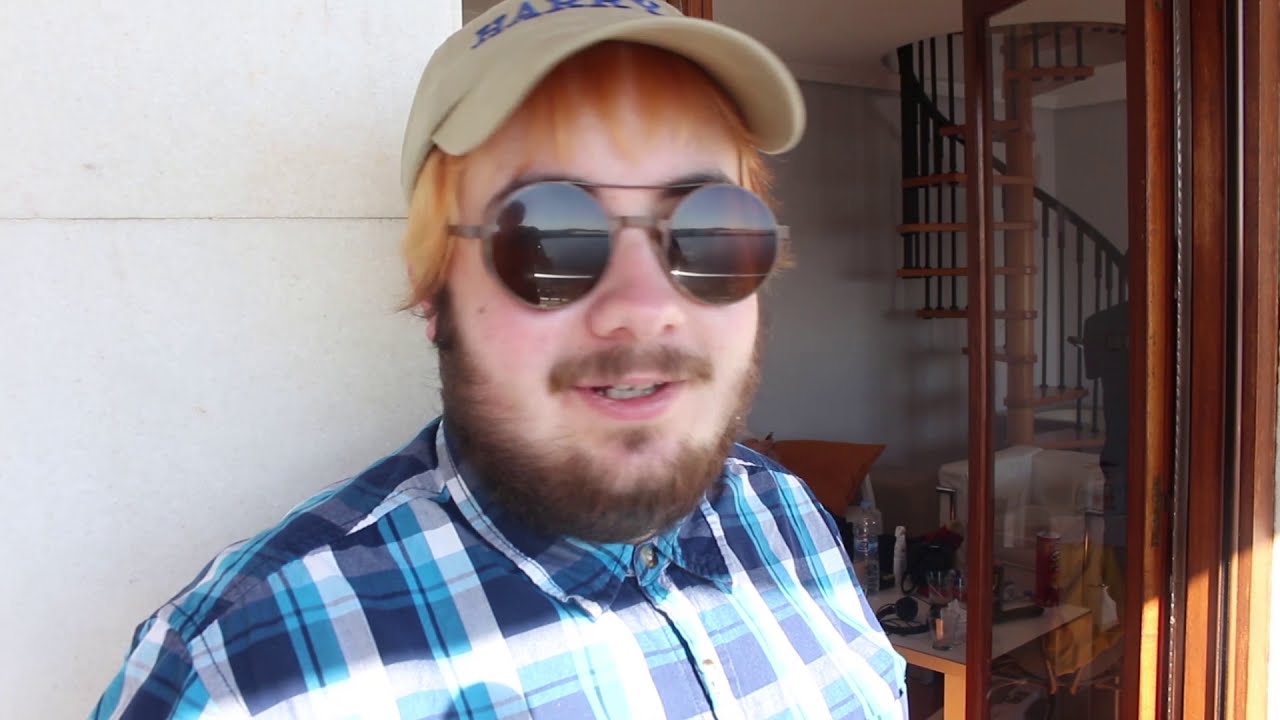The image features a pale-skinned, red-haired man with a scruffy brown beard and mustache, wearing a beige baseball cap and large, circular black sunglasses. Through the reflection in his sunglasses, someone taking the photo is visible. The man is dressed in a blue, turquoise, and white checkered shirt buttoned all the way up. He is standing outside, basking in sunlight, right by an open glass door that leads into a building. Inside, behind him and to his right, a stylish wooden spiral staircase is visible, along with a coffee table adorned with various objects, including a water bottle and possibly headphones. The man appears relaxed, enjoying the outdoors with a scenic view overlooking the sea.